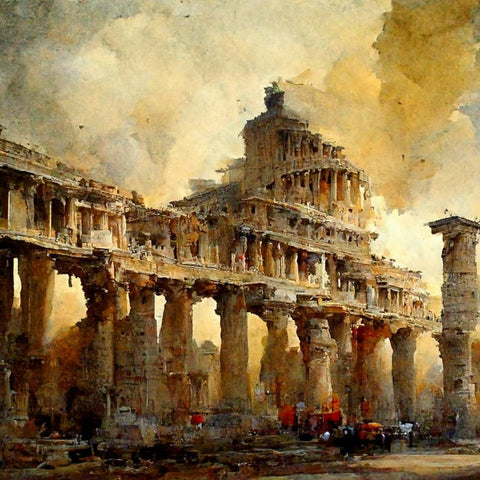This impressionist watercolor painting depicts ancient ruins reminiscent of Roman architecture, characterized by towering marble pillars and arched structures that evoke the grandeur of a once-mighty fortress now in various stages of disrepair. The primary structure, a multi-storied building with numerous arches, sits precariously atop the pillars, looking as though it could collapse at any moment. Below, indistinct figures and shapes, possibly representing vehicles, animals, or people in faded red and blue hues, add to the sense of disarray, while scattered wagons further suggest a scene of abandonment or conflict.

The atmosphere is heavy with smoke and cloud, painted in shades of gray, yellow, brown, orange, and blue, creating a somber mood. The gray sky above enhances the feeling of desolation. Though blurred and difficult to discern clearly, the painting conveys a vivid impression of a once-grand structure left in ruins, possibly ravaged by war or simply succumbing to the ravages of time. The use of muted colors and vague shapes adds to the painting's ethereal and haunting quality.